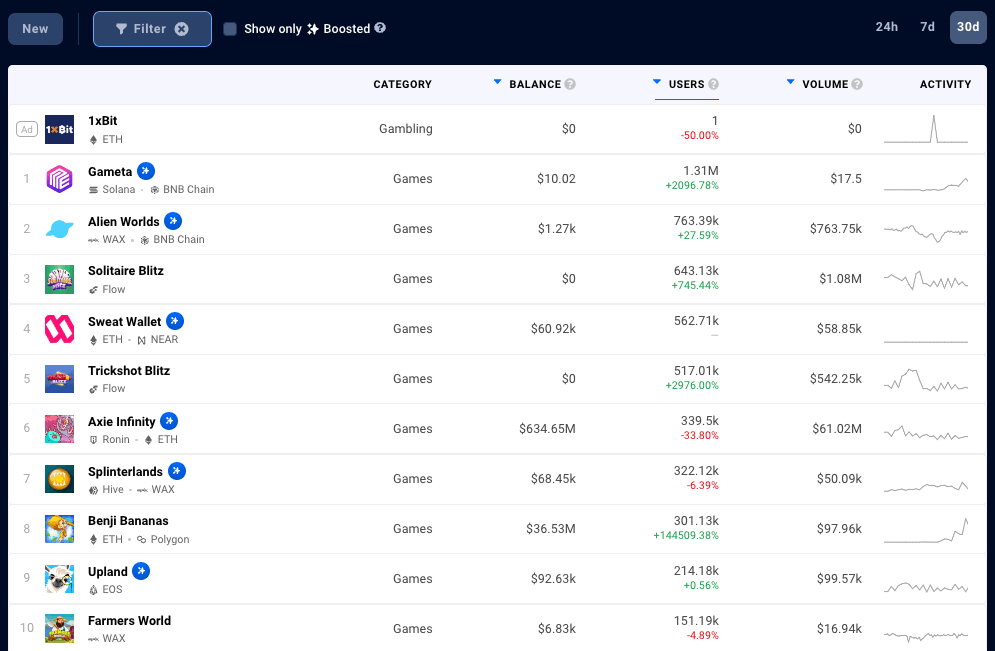This screenshot captures an interface filled with detailed analytics and data visualizations. At the top of the screen, there's a navigation bar with several interactive buttons. Starting on the upper left, the bar features a "New" button followed by a "Filter" button. There's also an empty checkbox with a label that reads "Show only," accompanied by a three-star AI symbol and the word "Boosted." Moving to the upper right corner, there are time frame filters allowing users to select data views for "24 hours," "7 days," or "30 days."

The main section of the screenshot is dominated by a comprehensive list sorted by various categories including gambling and gaming. Key metrics such as balances, users, volume, and activity are displayed in corresponding columns, providing a thorough overview of each category. Down the left side of the list are the names of different entities, each coupled with their corresponding rank and representative icons. The names listed are: 
1. Game Meta
2. Alien Worlds
3. Solitaire Blitz
4. Sweat Wallet
5. Trick Shot Blitz
6. Axie Infinity
7. Splinter Lands
8. Bingy Bananas
9. Upland
10. Farmer's World

Each of these entries is prominently numbered from 1 to 10, ensuring a clear and organized presentation of the data.